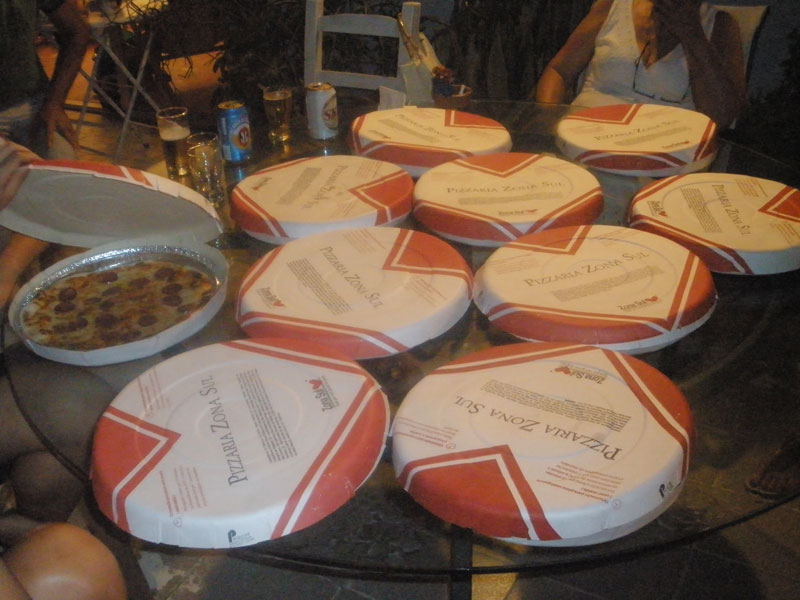The image depicts a nighttime outdoor setting with a large glass patio table holding several circular pizza containers. These containers resemble disposable tin pie plates, each covered with a round, red and white cardboard lid that says “Pizzeria Zona” in black writing. One of the containers is open, revealing a thin-crust pepperoni pizza inside. Around the table, a few people are visible, including a Caucasian woman in a sleeveless white top with glasses hanging around her neck and a partial view of her white tote bag. There are also beverages on the table, including clear glasses with yellow liquid, suggesting beer, and a blue can that might be Dr. Pepper. The scene is framed by some background plants and other indistinct human figures partially visible.